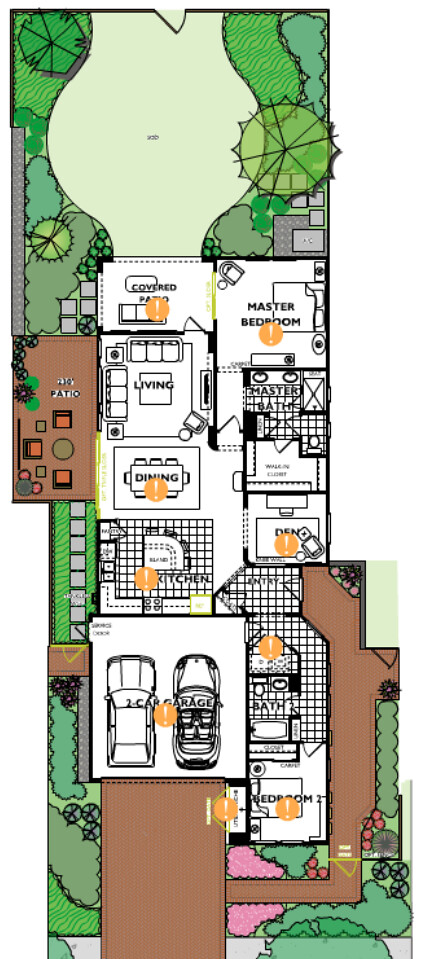This architectural drawing presents a detailed house plan viewed from the top, showcasing both the house and the surrounding yard. The house layout is marked with orange circles containing white exclamation marks in several rooms, but not all. The driveway, depicted as a brown rectangular area, is located towards the bottom left of the image. From the driveway, a brown pathway extends towards the right and then curves upward, indicating the route to the front garden and entrance.

The two-car garage is clearly labeled and leads to a potential front door. The floor plan inside the house identifies several rooms and areas: Bedroom 2, Bathroom 2, the entryway, a den positioned just behind the entry, and a kitchen situated prominently near the entry. Adjacent to the kitchen are the dining and living rooms, with additional details highlighting the master bath and master bedroom.

Two patios are depicted: a covered patio at the back of the house and an open patio to the left of the living and dining rooms. The backyard features a variety of greenery and a defined lawn area, creating a pleasant outdoor space.